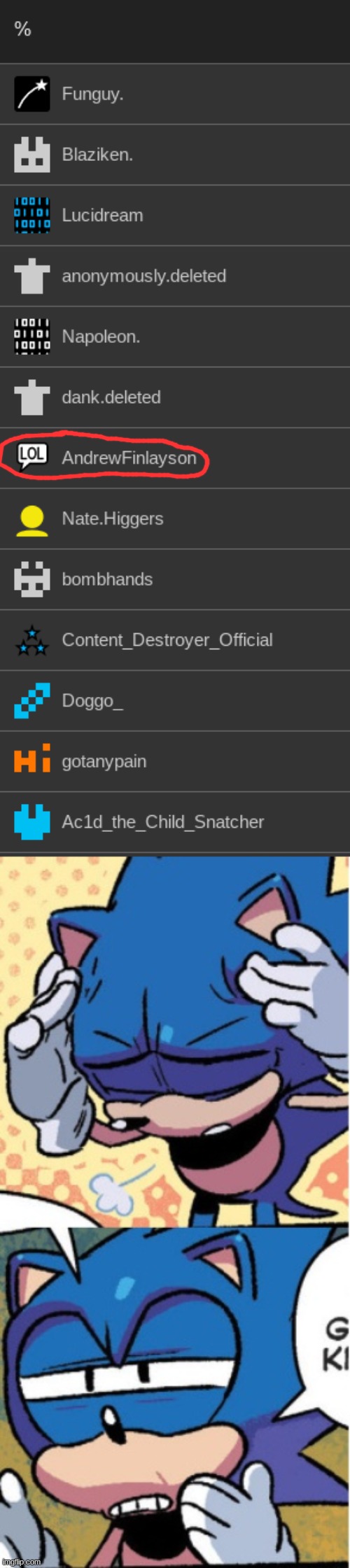In the top half of the image, a series of user icons accompanied by usernames can be seen. The usernames listed include Fun Guy, Blazekin, Lucid Dream, AnonymouslyDeleted, Napoleon, Dank.Deleted, Andrew Finalson, Nate Higgers, BombBirds, BombHands, ContentDestroyerOfficial, Doggo, GotAnyPainAcid, and TheChildSnatcher. Each user icon features unique imagery, such as a shooting star, a Lego-like face, a sequence of numbers and zeros, and a yellow emblem resembling a person, among others.

The lower portion of the image showcases two illustrations of Sonic the Hedgehog. In the first illustration, Sonic, the iconic blue hedgehog with white gloves, is depicted with his eyes closed, rubbing his temples as if in deep thought or frustration. In the second illustration, Sonic's eyes are partially open, and he appears to be saying something, although the text bubble containing his words is not visible.